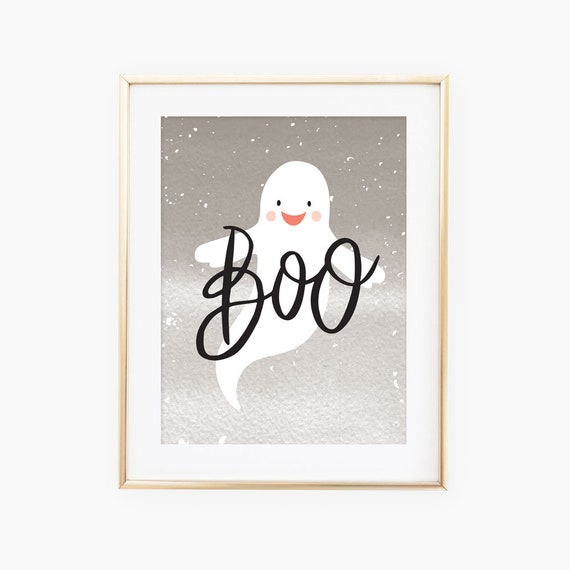The image depicts a framed piece of artwork hanging on a plain white wall. The frame is a thin, light brown or shiny light gold metal with a white matte border. The artwork itself features a cartoony ghost, centrally positioned, with a gradient gray sky as the background, darker at the top and lighter at the bottom, sprinkled with white specks resembling snow. The ghost is white with a curly, pointy tail, two arms stretched out, and a happy expression. It has wide black eyes, a reddish smiley mouth, and peach-colored rosy cheeks. Large black cursive text above the ghost reads "Boo."